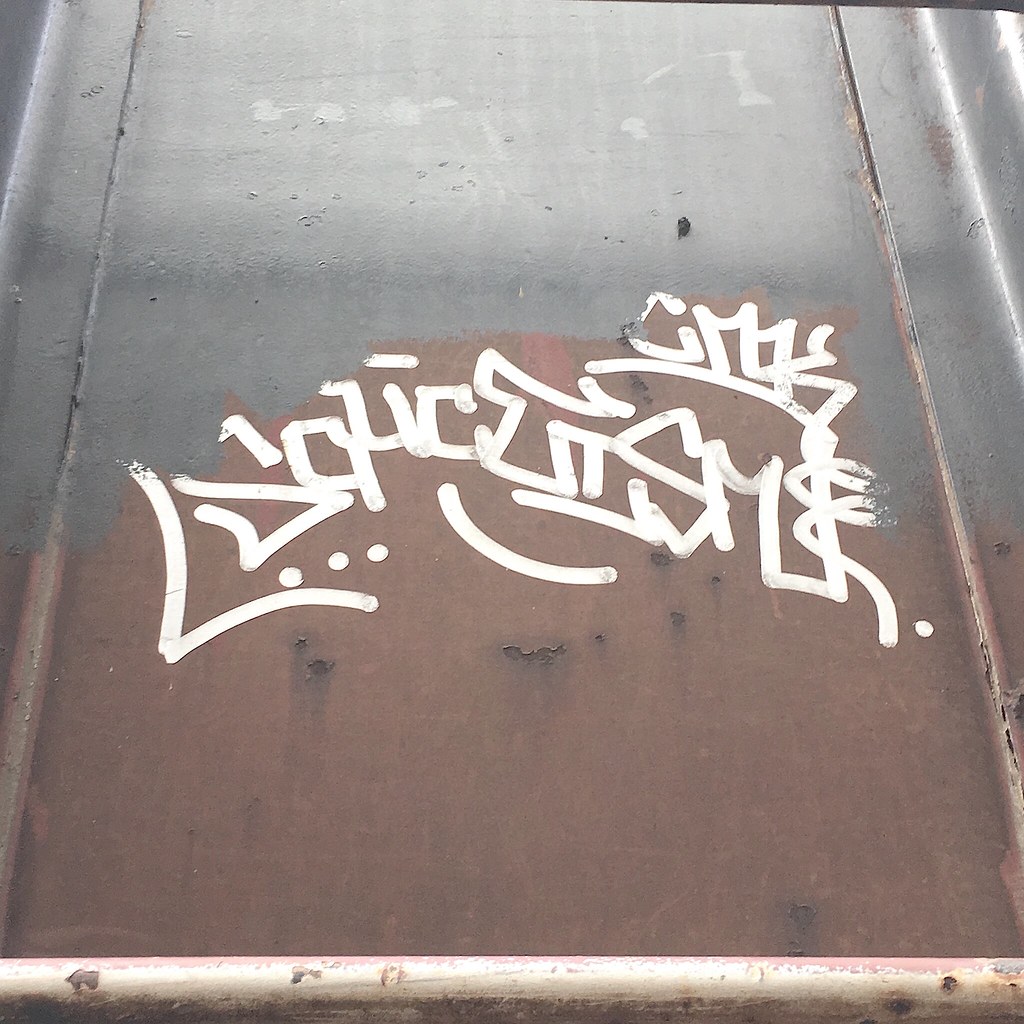The image is a vertical rectangular photograph of a corroded metal surface that appears either to be a wall or a large metallic object. The metal is primarily silver with patches that fade to a rust-like pink. Illuminated by light, it shines more on the right side and is darker on the left. The surface is mostly flat but has ridges along the sides and appears to be chipping in places, revealing its corroded nature. Across the bottom part of the metal, almost in the middle of the frame, there is white graffiti. The graffiti consists of various shapes and figures including what resembles a number one, a potential letter S, and a possible capital L, surrounded by dots and other random shapes. There also appears to be a metal railing at the very bottom of the frame, which is also chipped and runs horizontally from left to right.